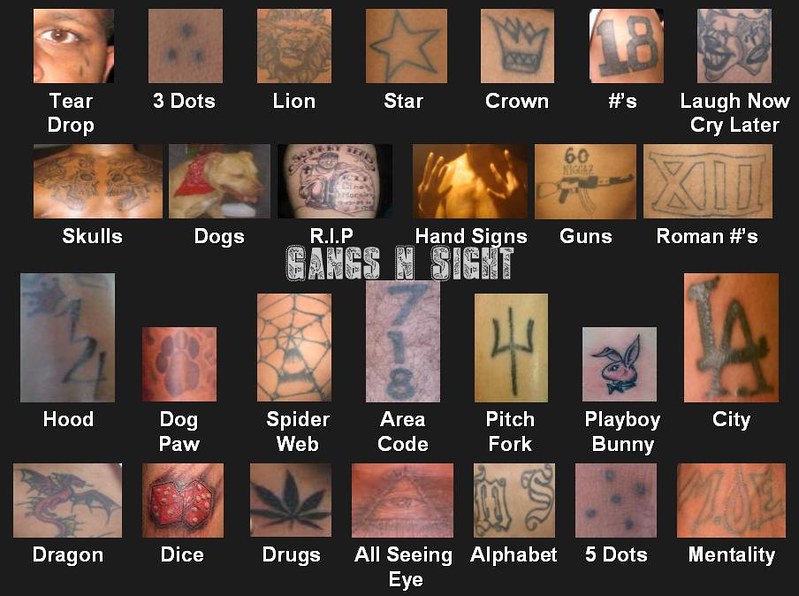The image titled "Gangs N Sight" is a detailed, rectangular collage set against a black background, composed of 24 individual images arranged in four rows. Each image vividly portrays various gang-affiliated tattoos and related symbology, accompanied by white text labels. The top row includes a teardrop tattoo under an eye labeled "Teardrop," a tattoo of three dots labeled "Three Dots," a lion tattoo labeled "Lion," a star tattoo labeled "Star," a crown tattoo labeled "Crown," the number 18 tattoo labeled "Numbers" accompanied by a hashtag, and a depiction of two clown faces with the phrase "Laugh Now Cry Later." 

The second row showcases tattoos and imagery such as skulls labeled "Skulls," a pit bull with a red bandana labeled "Dogs," an "R.I.P." tattoo featuring a figure leaning against a tombstone, hand signs labeled "Hand Signs," an automatic weapon tattoo labeled "Guns," and the Roman numeral XIII tattoo labeled "Roman Numbers."

Descending to the third row, the images present a tattoo partially obscured but labeled "Hood," a dog paw tattoo labeled "Dog Paw," a spider web tattoo labeled "Spider Web," a tattoo of 718 labeled "Area Code," a pitchfork tattoo labeled "Pitchfork," a Playboy bunny head tattoo labeled "Playboy Bunny," and an "LA" tattoo labeled "City."

The bottom row includes a dragon tattoo labeled "Dragon," red dice tattoo labeled "Dice," a marijuana leaf tattoo labeled "Drugs," an eye inside a pyramid labeled "All-Seeing Eye," a script tattoo of "MS" labeled "Alphabet," a tattoo of five dots labeled "Five Dots," and a blurry tattoo resembling "MOE" labeled "Mentality."